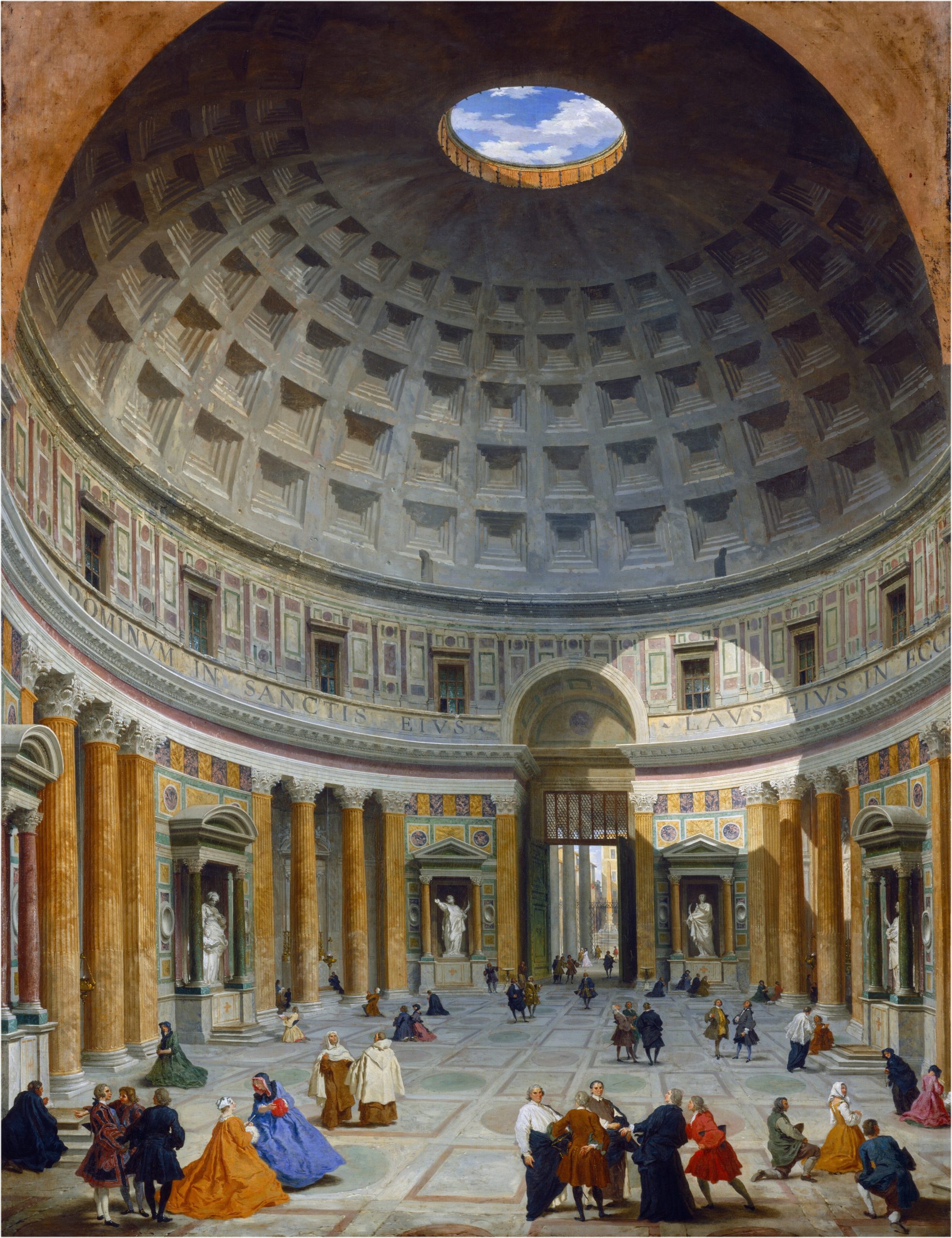The painting depicts the interior of a grand, ancient Roman-style building with an impressive stone dome. At the apex of the dome is a circular open skylight, showcasing a view of the blue sky and clouds. Light from the skylight cascades down, illuminating sections of the interior walls. The dome itself and the mid-floor are adorned with numerous cut-in indentations and a series of windows, respectively. 

The main floor is intricately ornate, featuring multiple alcoves that house marble statues. These statues are nestled between numerous orange-brown columns that add to the architectural grandeur. The scene is bustling with people from various walks of life, all dressed in elaborate, period-specific attire. Among them are individuals in vibrant blue and orange gowns, men in red and dark blue suits, and religious figures such as nuns. One notably corpulent man stands out in the foreground, attired in black or blue pants and a white shirt. The overall atmosphere evokes the timeless elegance and grandiosity of a bygone era.